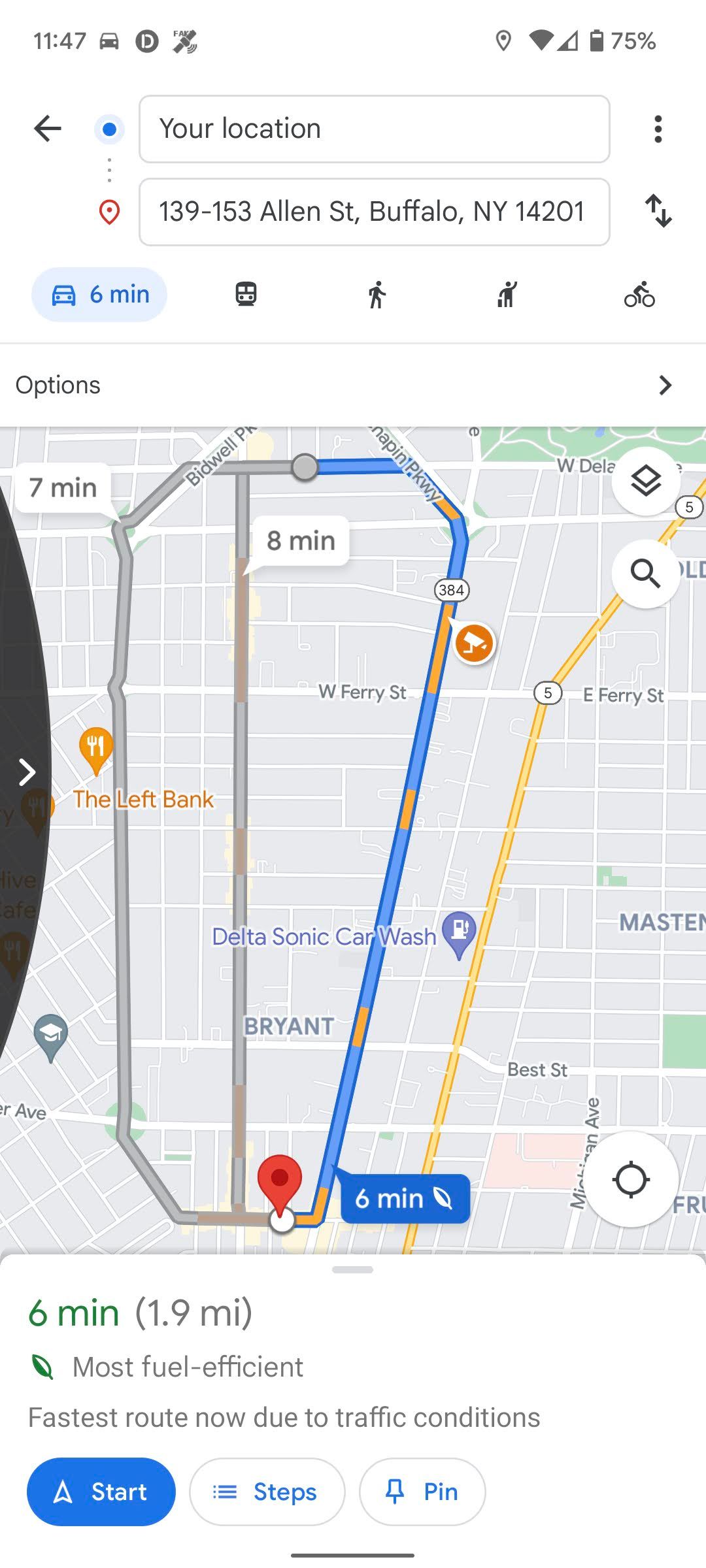A detailed screen capture of a smartphone reveals that it's 11:47 AM with the battery 75% charged. The screen shows a navigation app where the search bar indicates the current location as 139-153 Allen Street, Buffalo, New York, zip code 14201. Displaying a small map with nearby roads, a red pin marks a specific point, suggesting either the user's present location or destination. Below the map, the app advises that the most fuel-efficient and fastest route, given the current traffic conditions, is a 1.9-mile journey taking approximately six minutes. The user appears to be in the process of plotting their next move using the app.